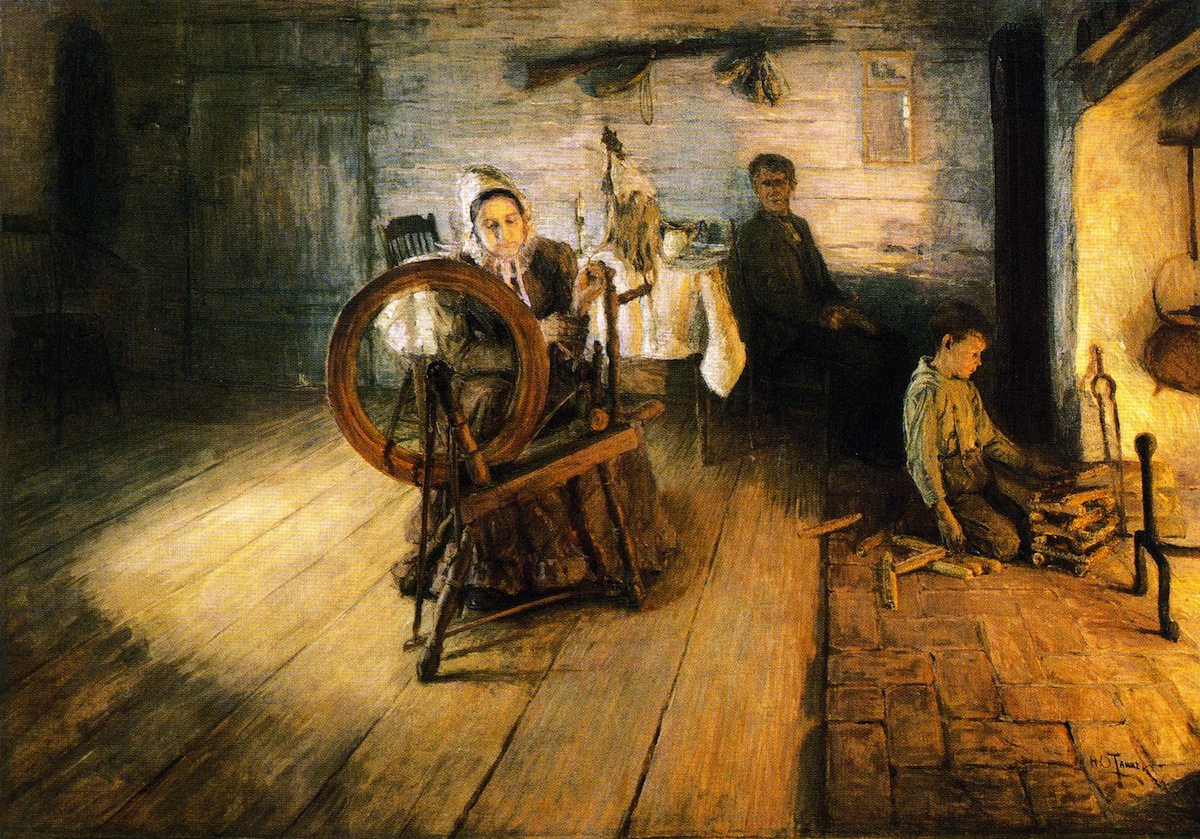The painting depicts a detailed colonial-era scene set inside a rustic wooden cabin. Central to the composition is a woman, dressed in a bonnet and long dress, seated at a wooden spinning wheel, diligently weaving threads. To her left, a young boy in cloth overalls and a long-sleeve shirt crouches by a brick-lined fireplace, holding a piece of wood poised to stoke the fire. The warm glow from the fireplace casts light on the wooden panel floors and surrounding area.

In the background, partially shrouded in shadows, a man in a suit sits on a chair against a light-colored wall. He glances over his right shoulder at the woman, who remains focused on her spinning wheel. Nearby, against the same wall, a shotgun is mounted, and a white-clothed table stands behind the man, accompanied by an empty chair. On the opposite side of the room, there is another table, this one brown and uncovered.

The room exudes a cozy yet utilitarian atmosphere, with the wooden door and hanging jacket contributing to the lived-in feel. The intricate details of the painting effectively capture a moment from a bygone era, showcasing the simplicity and craftsmanship of colonial life.